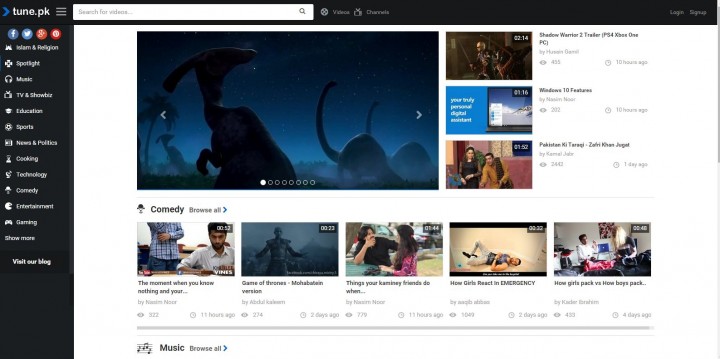The webpage, identified by its header "toon.pk," features a sleek interface with a blue arrow and a search bar that reads "search for videos" accompanied by a grey magnifying glass icon. Users can refine their search to either "videos" or "channels" through a handy toggle option. Running along the right side of the page is an extensive list of categories, arranged as follows: Islam and Religion, Spotlight, Music, TV and Showbiz, Education, Sports, News and Politics, Cooking, Technology, Comedy, Entertainment, and Gaming. A "Show More" link is available for additional categories, along with the "Visit Our Blog" button for further engagement.

Social media icons are conveniently located for easy sharing and connectivity. The main page prominently displays a video, likely depicting several large animals that resemble dinosaurs against a starry night sky. Adjacent to this, a "Shadow Warrior 2" trailer for PS4, Xbox One, and PC is featured, showcasing video game characters. A "Windows 10 Features" video, running for 1 minute and 16 seconds, is also available. Additionally, the Comedy section boasts a variety of engaging thumbnail images and music clips. The overall design of the webpage is clean and bright, set against a white background adorned with diverse and vibrant images.